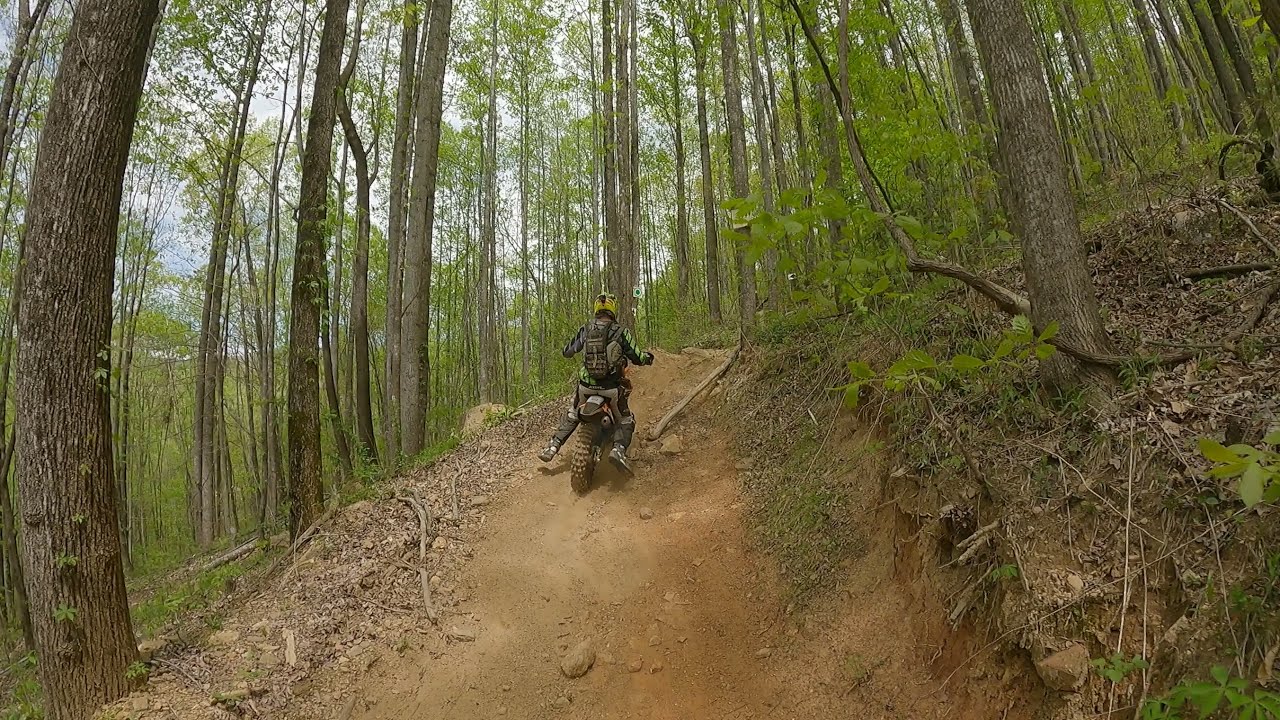In this clear, color photograph taken during the day, an individual is captured navigating a steep dirt path on a dirt bike. The rider, seen from behind, wears full protective gear, including a yellow helmet, a thick jacket, gloves, shin guards, and a backpack. The steep trail ascends both forward and to the right, stretching from the bottom left to nearly the top right of the image, emphasizing the challenging incline. Flanking the dirt path are numerous trees, varying in thickness, with narrow trunks and sparse green foliage, indicative of a season like early spring. The terrain, both on and off the trail, is predominantly dirt with coarse roots, sticks, and a scattering of leaves, underscoring the rugged outdoor setting on this partly cloudy day.